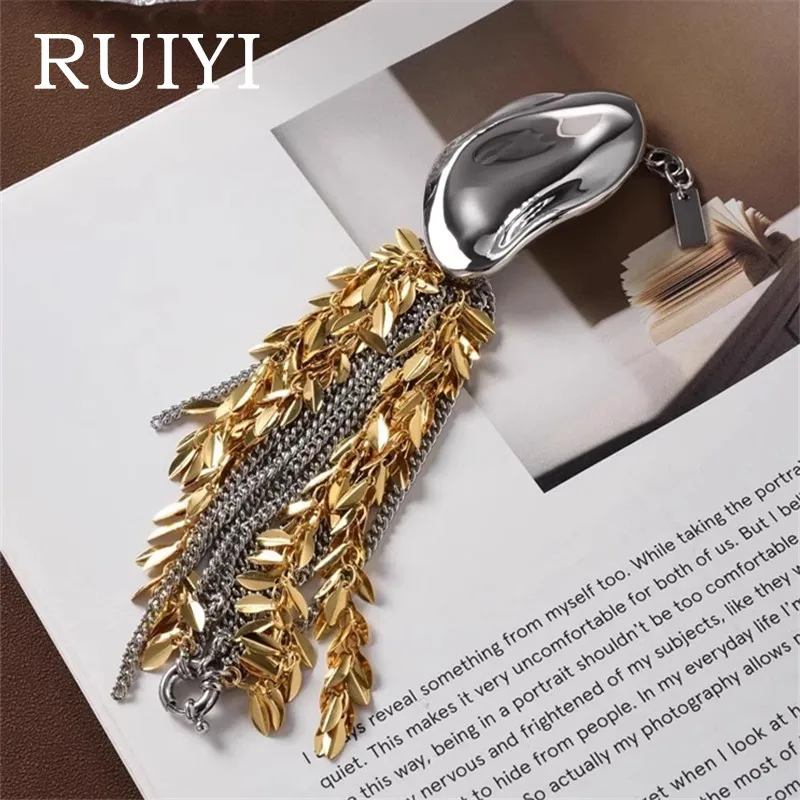The photograph captures an artistic scene where a metallic charm, resembling either a bookmark or a piece of jewelry, rests upon the pages of an open book. The charm consists of a silver oval top adorned with short chains and a small, illegible tag. From the bottom, several chains cascade, featuring both silver links and gold leaves. The open book is positioned on a white surface, with a superimposed image of another open book on a white table, creating a layered, "Inception-like" effect. In the top left corner of the white piece of paper, the word "RUIYI" is prominently displayed in all caps. Toward the bottom of the image, partially visible text from the book reads: "I always reveal something from myself, too, while taking the portrait... quiet. This makes it very uncomfortable for both of us, but I bet, this way, being in a portrait shouldn't be too comfortable... nervous and frightened of my subjects like they... to hide from people. In my everyday life, I'm... so actually, my photography allows... when I look at... the most of..." The scene is set against a dark brown carpet, adding depth to the composition. The fresh-looking pages of the book stand out starkly against the darker background, enhancing the photograph's textured and multi-layered aesthetic.